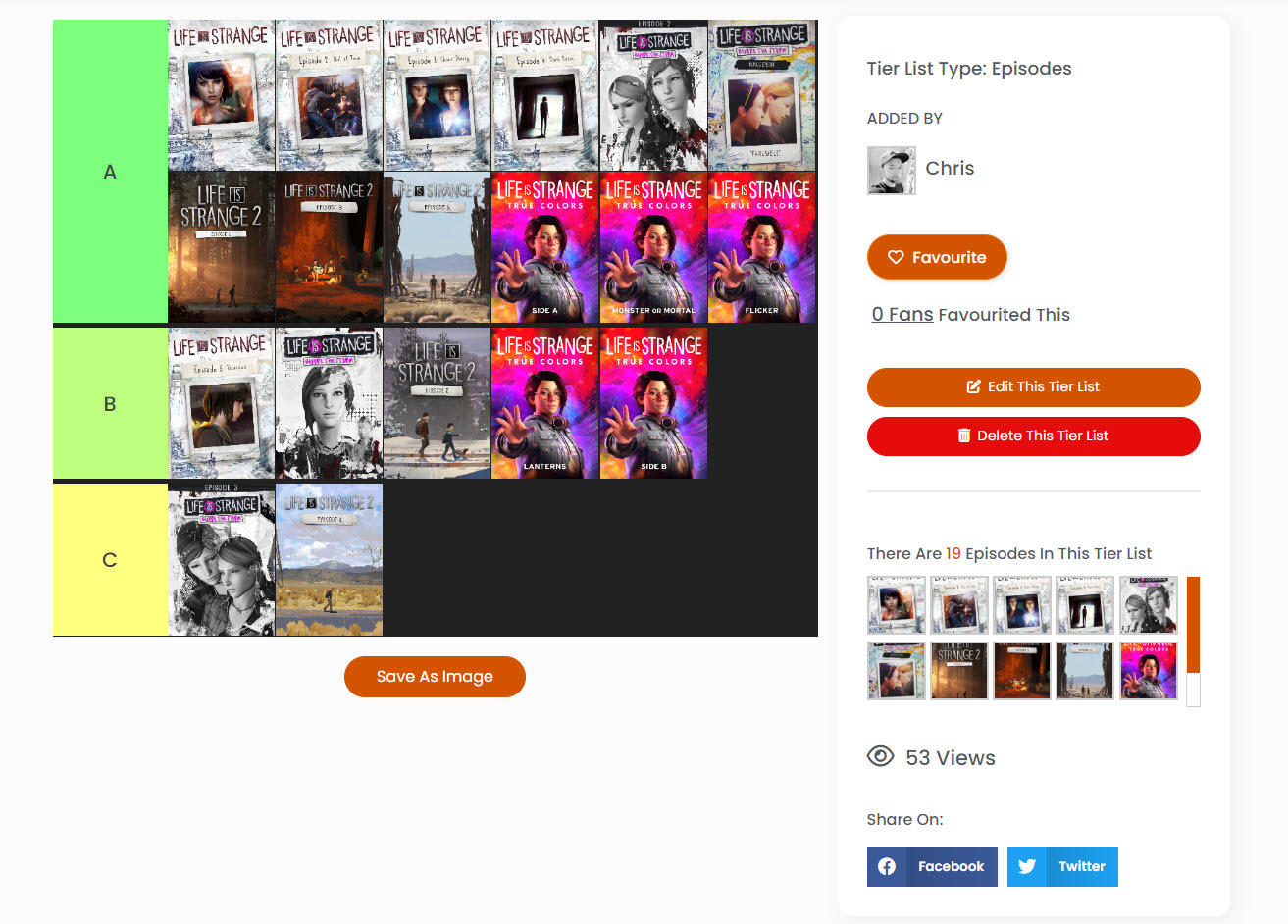Here is the cleaned-up and detailed caption:

"A meticulously organized tier list created by Chris, categorizing 19 episodes from the 'Life is Strange' video game series. The top of the tier list features a control bar with options to add, edit, or delete tiers, and displays a total of 53 views along with buttons to share on Facebook and Twitter. Additionally, there's a 'Save Image' button located to the right of the view count.

The tier list is color-coded, with 'A' tier episodes highlighted in green, 'B' tier in lighter green, and 'C' tier in yellow. It showcases various episodes from the 'Life is Strange' games, with many featuring female characters prominently displayed. Notable inclusions are episodes with characters possessing varying hair colors such as brown and gray, along with a couple of episodes that depict male characters from a distance.

Under this system, 12 episodes are ranked in the 'A' tier, 5 in the 'B' tier, and 2 in the 'C' tier. The list includes episodes from titles like 'Life is Strange,' 'Life is Strange 2,' and other installments from the franchise. Each episode image provides distinct visual cues, often highlighting the series' prominent female protagonists."